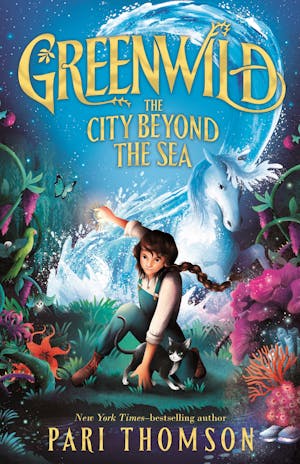The cover of the children's book "Greenwild, the City Beyond the Sea" by New York Times bestselling author Perry Thompson, showcases a captivating scene filled with fantastical elements. Dominating the artwork is a young, androgynous figure with a long brown braid, clad in green overalls and a white shirt, crouching in an action pose reminiscent of a Marvel superhero. Beneath the child rests a black and white cat, adding a touch of companionship to the scene. The backdrop is a vibrant, digitally illustrated collage blending various elements: a swirling massive wave of water, a prancing white horse (or potentially a unicorn) integrated into the wave, and a night sky transitioning into lush grassy land. Surrounding the central figures are an array of colorful, fantasy-like plants, complete with purple flowers, butterflies, and a green parrot. Further down, the scene transforms into a marine environment with elements such as anemones and starfish, enveloping the adventurous spirit of the cover. Above the child's head, in bold gold print, is the title "Greenwild, the City Beyond the Sea," while at the bottom, Perry Thompson’s name is proudly displayed, affirming their acclaim.